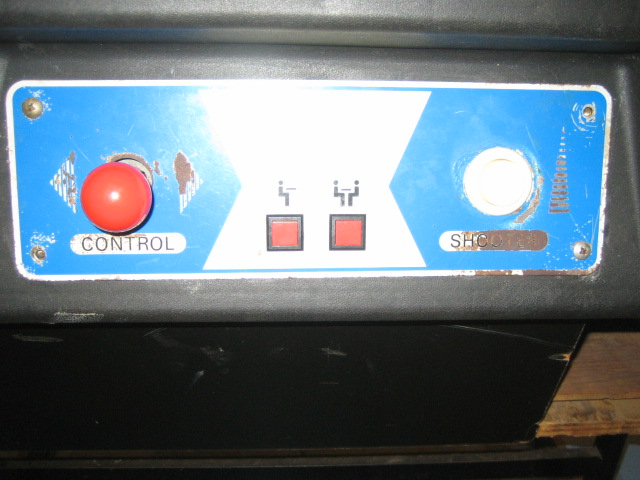The photo features a control panel of a vintage sit-down arcade game, showcasing its worn-out and well-used state. The control panel is decorated with a faded blue background and a silver border. On the left side, there's a red ball joystick labeled "control," flanked by a faded left-pointing arrow and an almost indiscernible right-pointing arrow. In the center of the panel are two square red buttons: the left button is for single-player mode, featuring an illustration of a person sitting alone, while the right button is for multiplayer mode, illustrated with two people sitting together. On the far right is a white button labeled "shooter," though the text is heavily worn and barely legible. The control panel sits atop a black or gray arcade machine, adding to the overall nostalgic and aged aesthetic.